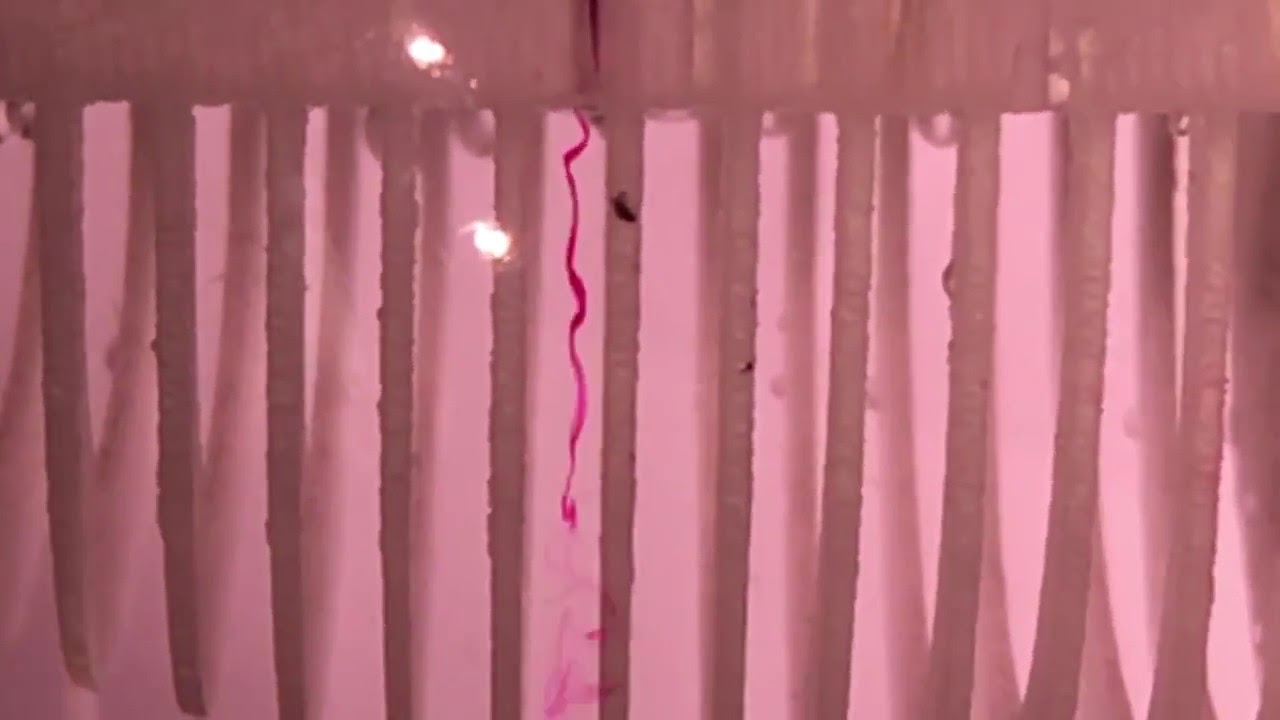This is a horizontal rectangular image that appears to be an abstract painting dominated by various shades of pink. The composition features numerous tall, skinny rectangles in lighter pink hues arranged against a darker pink background, resembling rectangular birthday candles with square tops, some even suggesting a flame. Toward the left side and near the top of one rectangle, there are two bright yellow spots that could be light reflections. In the center, one of the rectangles has a fuchsia-pink squiggly line running down about two-thirds of its height, with a darker rectangular shape positioned above it. The image has a pixelated, blurry quality, suggesting it might be a screenshot or a low-resolution photograph, hence some details appear indistinct. There are approximately 20 vertical columns that make the structure look somewhat mechanical or plastic, and in the top central part of the painting, there are additional white dots that could signify more light reflections. A noticeable black dot on one of the columns might be a spot of dirt or an imperfection in the image.